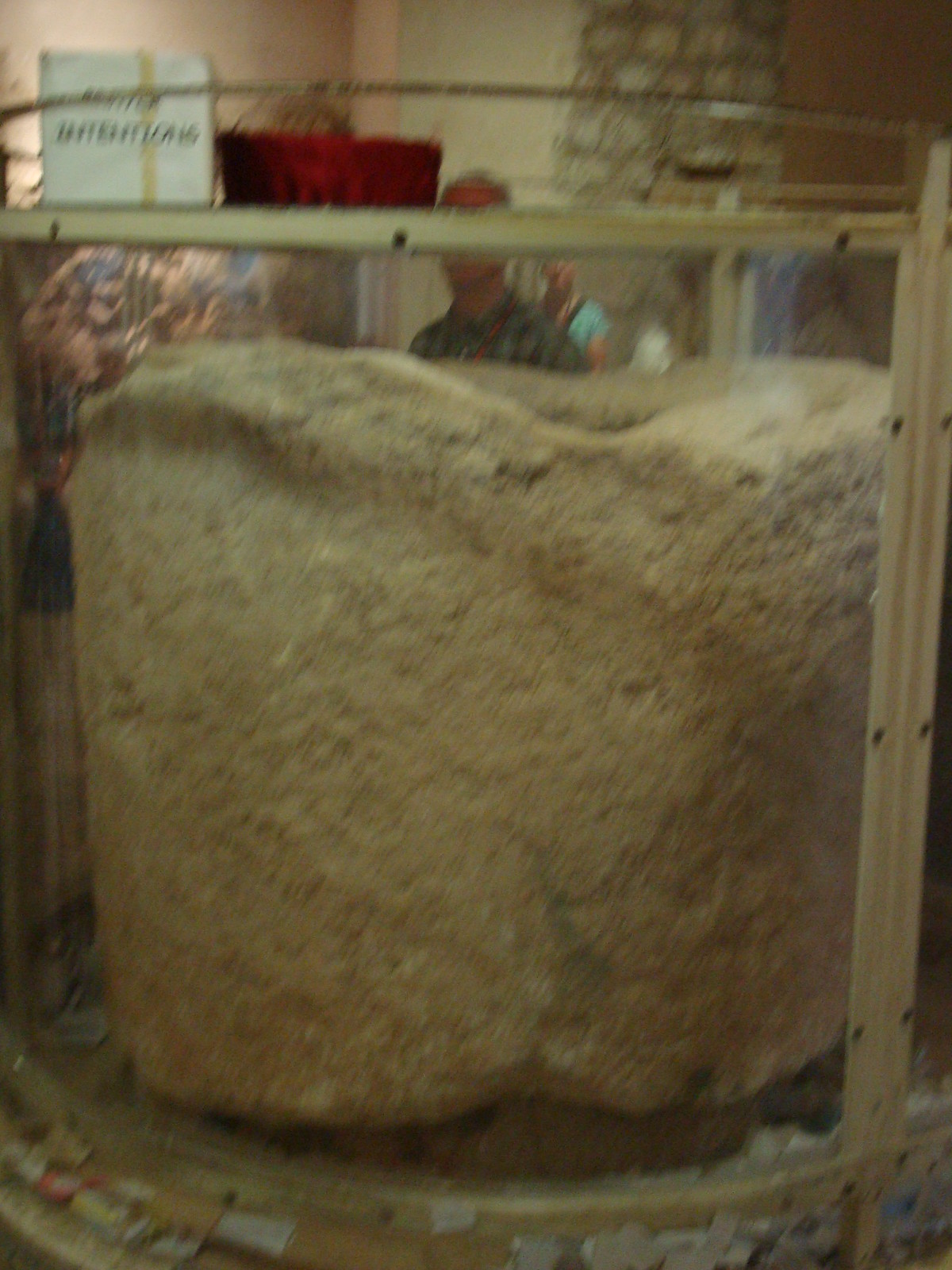The photograph captures a large, cylindrical, sand-colored stone meticulously encased within a round glass and metal display case, accented with gold trim. The case sits in an indoor setting, suggested by the blush-colored painted wall and the primitive brick-and-concrete pillar visible in the background. On top of the display, a white sign with indistinguishable letters is prominently mounted. In the background, slightly out of focus, stands a man donning a plaid shirt and a woman in a light blue short-sleeved shirt with a strap across it. The man observes the stone intently, hinting at the stone's significance, likely as a museum artifact. The stone itself, reminiscent of a large footstool in size, appears smooth yet subtly textured, with a possible hole descending from its top center. A red basket is also visible atop the display case.